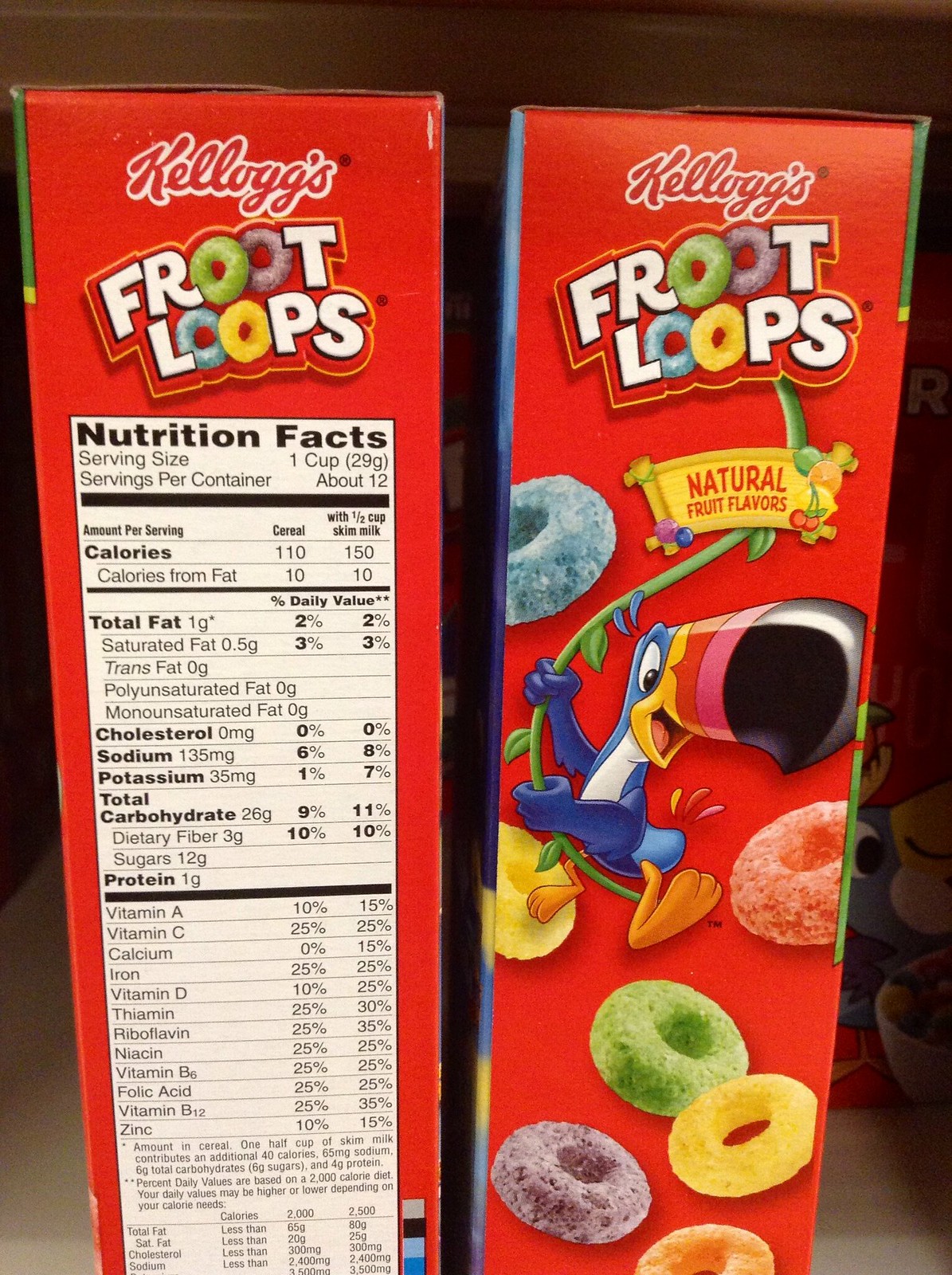This photograph features two side-by-side packages of Kellogg's Froot Loops cereal, captured from the side view rather than the front. The focus is on the side panel of the box on the right, which prominently displays the colorful Kellogg's Froot Loops logo along with the text "Natural Fruit Flavors." Central to this side panel is an illustration of the iconic Toucan Sam, depicted swinging from a vine with vibrant Froot Loops cereal pieces scattered above and below him. His beak is pointed to the right, directing attention across the image. The side panel of the left-hand package showcases the Nutrition Facts label clearly, a white rectangle outlined in black, detailing the nutritional information in crisp, black lettering. Above this label, the Kellogg's brand name is written in its characteristic red font, accompanied by the Froot Loops logo. To the right of these features, the red back of the cereal box is partially visible.